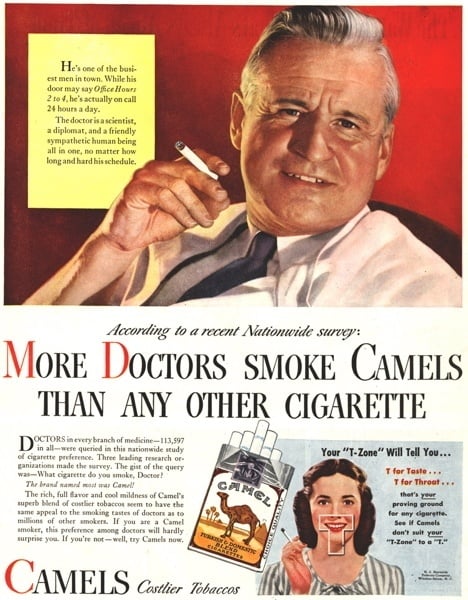This vintage Camel Cigarettes advertisement features an older, content-looking white man with gray, slicked-back hair, dressed in a white shirt and black tie. He is lounging in a chair, facing slightly to the left, and holding a cigarette in his right hand against a red background. Above him, a yellow box contains text extolling his dedication and hard work, stating he is one of the busiest men in town, available 24 hours a day despite his office hours being officially from two to four. Black and red text highlights a survey stating, "More doctors smoke Camels than any other cigarette," with the prominent letters "M" and "D" in red. The lower section of the image features a smiling woman with brown hair and red lipstick, dressed in a white and gray striped top, holding a cigarette. She is positioned next to a pack of Camel Cigarettes and the text, "Your T-zone will tell you: T for taste and T for throat." The cursive script in the bottom left corner reads "Camel Cigarettes" followed by "Costlier Tobaccos" in black print with the first "C" in red, enhancing the nostalgic appeal of this advertisement.